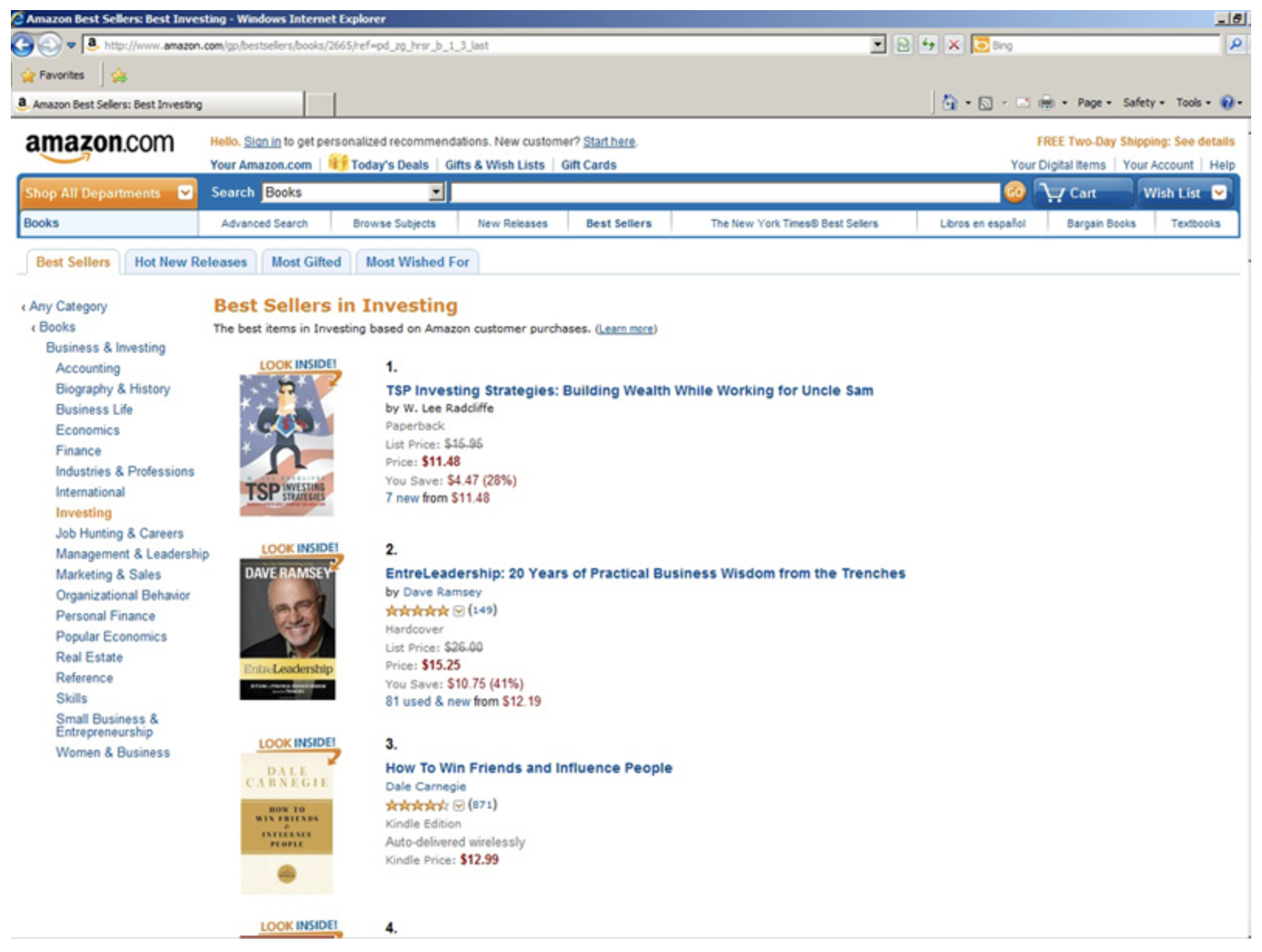In this detailed screenshot from Amazon.com, the layout showcases the vibrant options available for book shopping. The top left corner displays the Amazon logo, while beneath it is a navigation tab labeled "Shop All Departments," with a focused subcategory of "Books." Directly adjacent to this is a search bar, followed by a cart button and a wishlist button for easy user access.

Centered above the main content area are several interactive tabs: "Advanced Search," "Browse Subjects," "New Releases," "Best Sellers," "The New York Times Best Sellers," "Libraries in Spanish," "Bargain Books," and "Textbooks." The highlighted tab is "Best Sellers," indicating that the user is currently viewing this category. Other selectable options include "Hot New Releases," "Most Gifted," and "Most Wished For."

Within the "Best Sellers" section, the results pertain to investing books. Displayed prominently at the top of the list:

1. "TSP Investing Strategies: Building Wealth While Working for Uncle Sam"
2. "EntreLeadership: 20 Years of Practical Business Wisdom from the Trenches"
3. "How to Win Friends and Influence People"

The fourth book’s title is partially cut off, leaving only the ranking number visible at the bottom. This structured and informative display provides a snapshot of popular investing literature available to Amazon users.